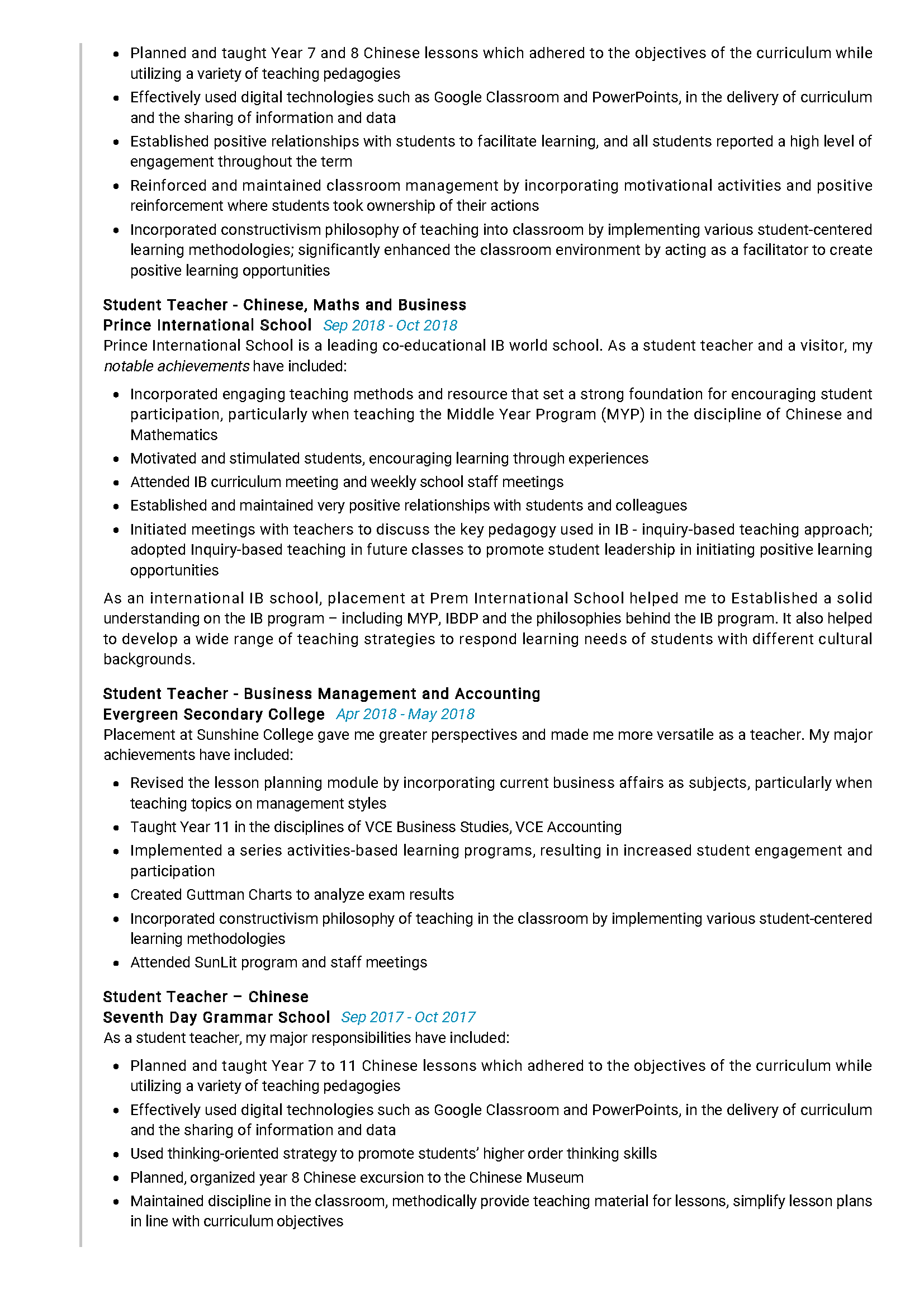This screenshot showcases a resume focused on various teaching roles with an emphasis on Chinese language instruction. The excerpt opens mid-sentence, detailing tasks from a previous job. Specifically, the individual planned and executed Chinese lessons for Year 7 and Year 8 students according to curriculum objectives, employing diverse teaching methodologies.

Following this, the resume features a section highlighting the individual's role at Prince International School from September 2018 to October 2018. It is noted that Prince International School is a leading co-educational IB World School. Here, the person served as a student teacher for Chinese, Maths, and Business, achieving several notable milestones (listed in bullet points below the description).

The subsequent section describes a position at Evergreen Secondary College where the individual worked as a student teacher in Business Management and Accounting from April 2018 to May 2018. This placement is noted to have offered valuable experiences, enhancing the individual's versatility as a teacher. Key achievements during this tenure are also itemized in bullet points.

Another teaching stint is detailed at Seventh Day Grammar School from September 2017 to October 2017, where the individual served as a student teacher in Chinese. Responsibilities for this role, much like the others, are clearly outlined in bullet points to provide a thorough understanding of the tasks undertaken during this period.

All dates are prominently displayed in blue, providing a clear timeline of the individual's teaching experience across different institutions.